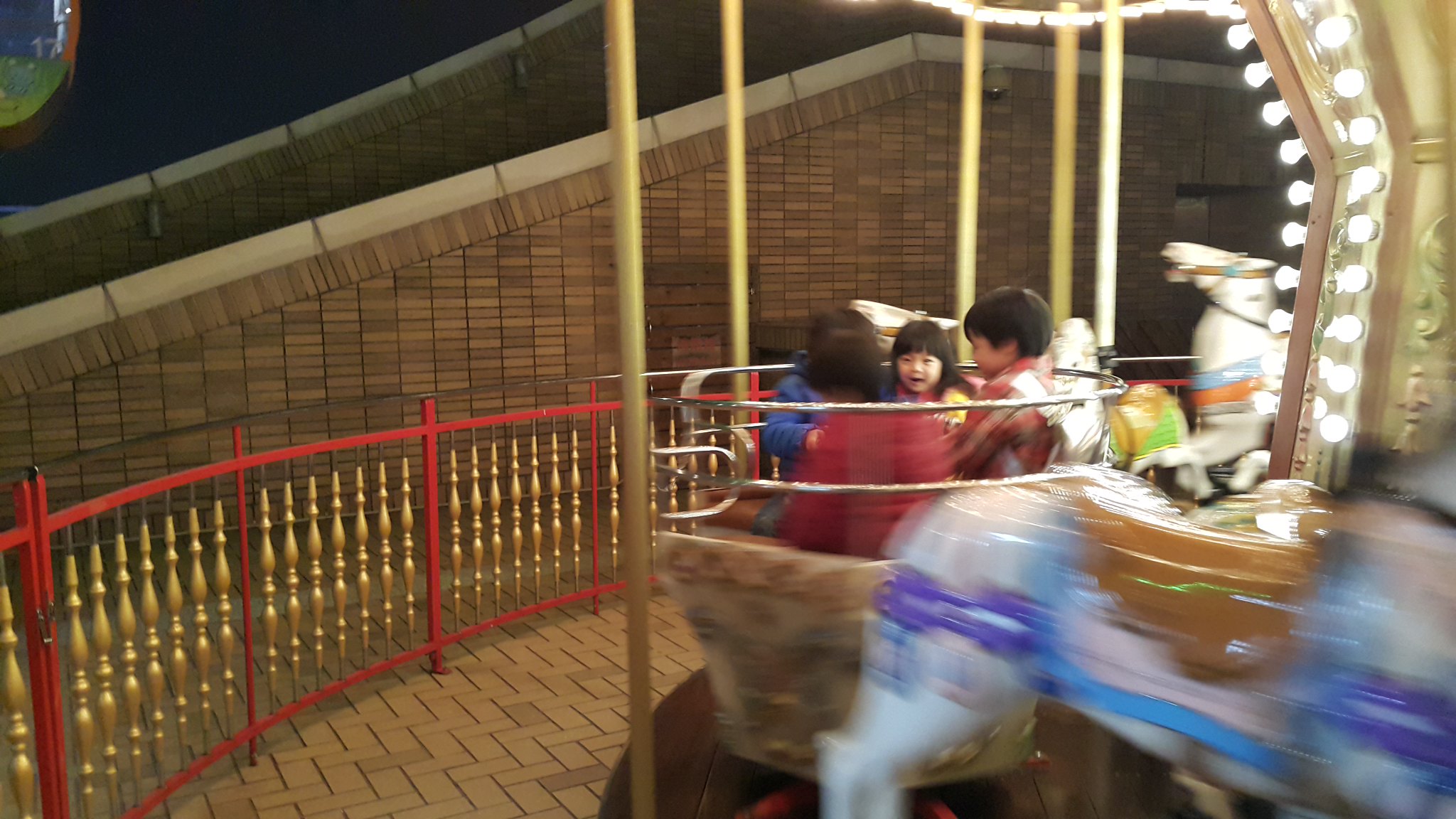This photograph captures a dynamic amusement park scene centered on a carousel ride in motion. The focal point is a group of four children, including a smiling little girl and a boy sitting next to her, nestled together inside a teacup-shaped compartment that spins as the carousel operates. The bright, shiny surface in the foreground appears slightly blurred, underscoring the motion. Surrounding the ride is a red decorative fence adorned with gold accents, ensuring safety by cordoning off the area. In the background, a stone or brick wall can be seen, possibly with steps leading to another level of the park. The image effectively conveys the joy and excitement of the children amidst the ornate and lively surroundings of the amusement park.